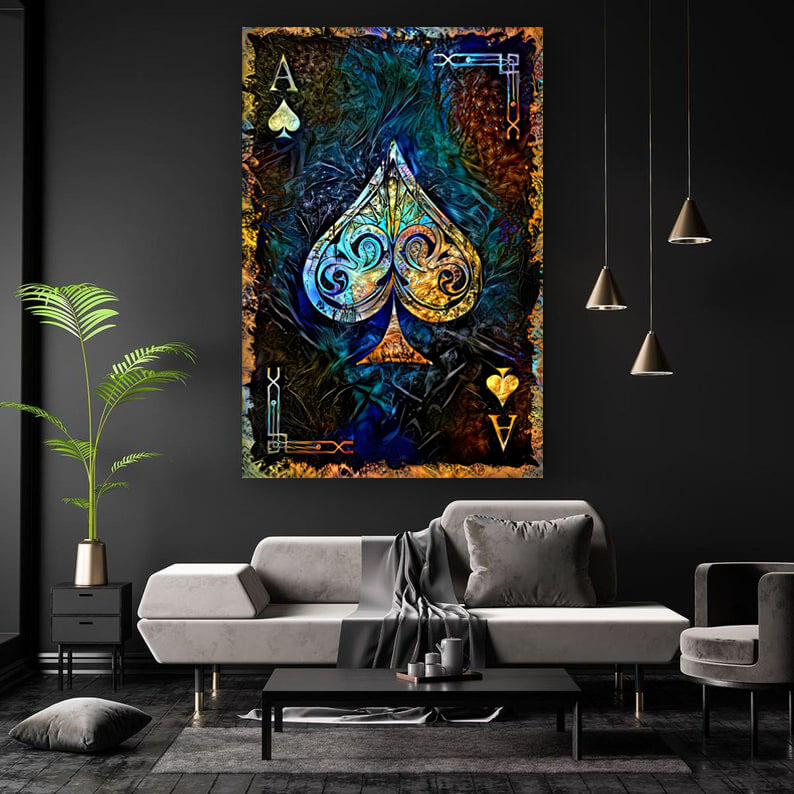This is a highly detailed photograph of a contemporary living room dominated by dark gray and black hues. The focal point is a large, vibrant artwork on the wall, depicting an Ace of Spades card with an intricate, colorful design featuring shades of blue, red, orange, yellow, and gold. The background of the artwork is a patterned blend of blues and greens.

The room has black walls and a gray and black tile floor, creating a sleek, modern atmosphere. In the center of the room is a distinctive modern gray couch with an uneven, stepped backrest design. Draped over the couch is a gray throw blanket, and there is a matching gray pillow on the couch and another pillow on the floor.

To the left of the couch is a small black table with two drawers, featuring black handles. On top of the table is a metallic silver pot holding a green fern-like plant. A modern round gray stool and a contemporary rounded gray chair are situated to the right of the couch.

Three copper-colored, cone-shaped hanging lights descend at varying lengths from the ceiling on the right side of the room. In front of the couch, there is a black coffee table adorned with a few cylindrical items, possibly candles. A black rug lies beneath the coffee table, tying the room's contemporary and minimalist design together.